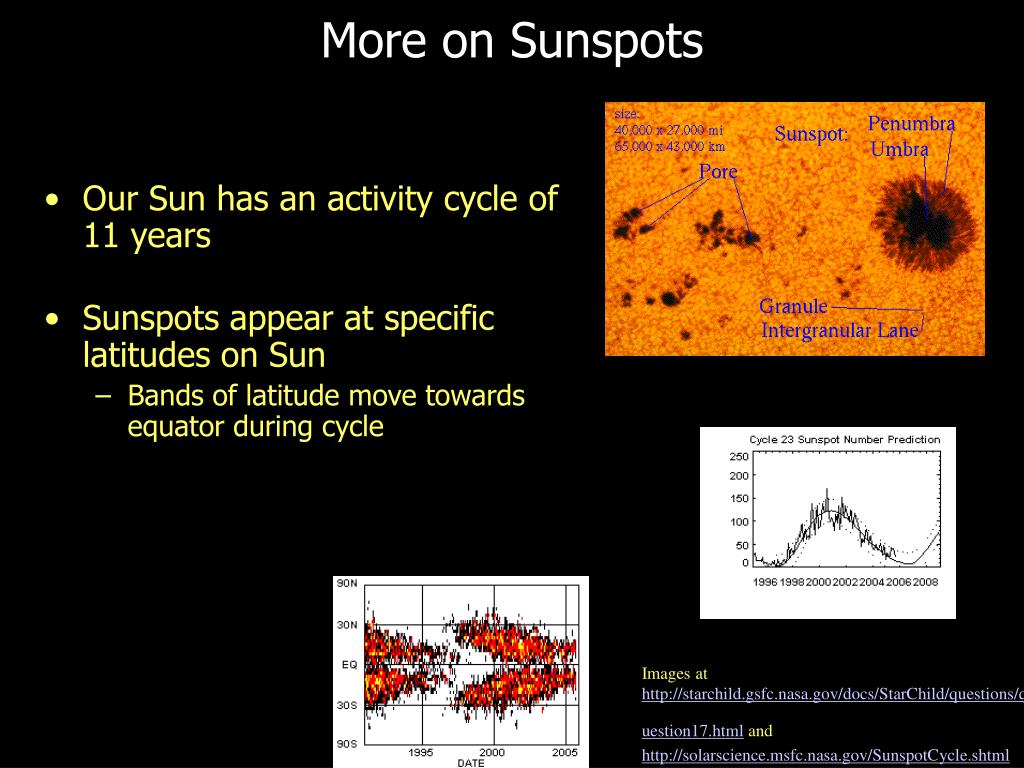This image resembles a PowerPoint presentation slide with a black background, titled "More on Sunspots" in white text at the top center. Below the title, two bullet points in yellow text on the left side of the slide provide key information: "Our Sun has an activity cycle of 11 years," and "Sunspots appear at specific latitudes on the Sun. Bands of latitudes move towards the equator during the cycle." 

On the right side of the slide, an orange diagram illustrates sunspots on the surface of the Sun. This diagram includes small black spots, labeled as pores on the left, and a larger area of black sparks with a brown edge on the right. Below this diagram is a graph titled "Cycle 23 Sunspot Number Prediction," showing the frequency and distribution of sunspots over time. The overall layout, color scheme (including white, black, orange, red, and yellow), and style suggest it is designed for an educational or informational presentation.